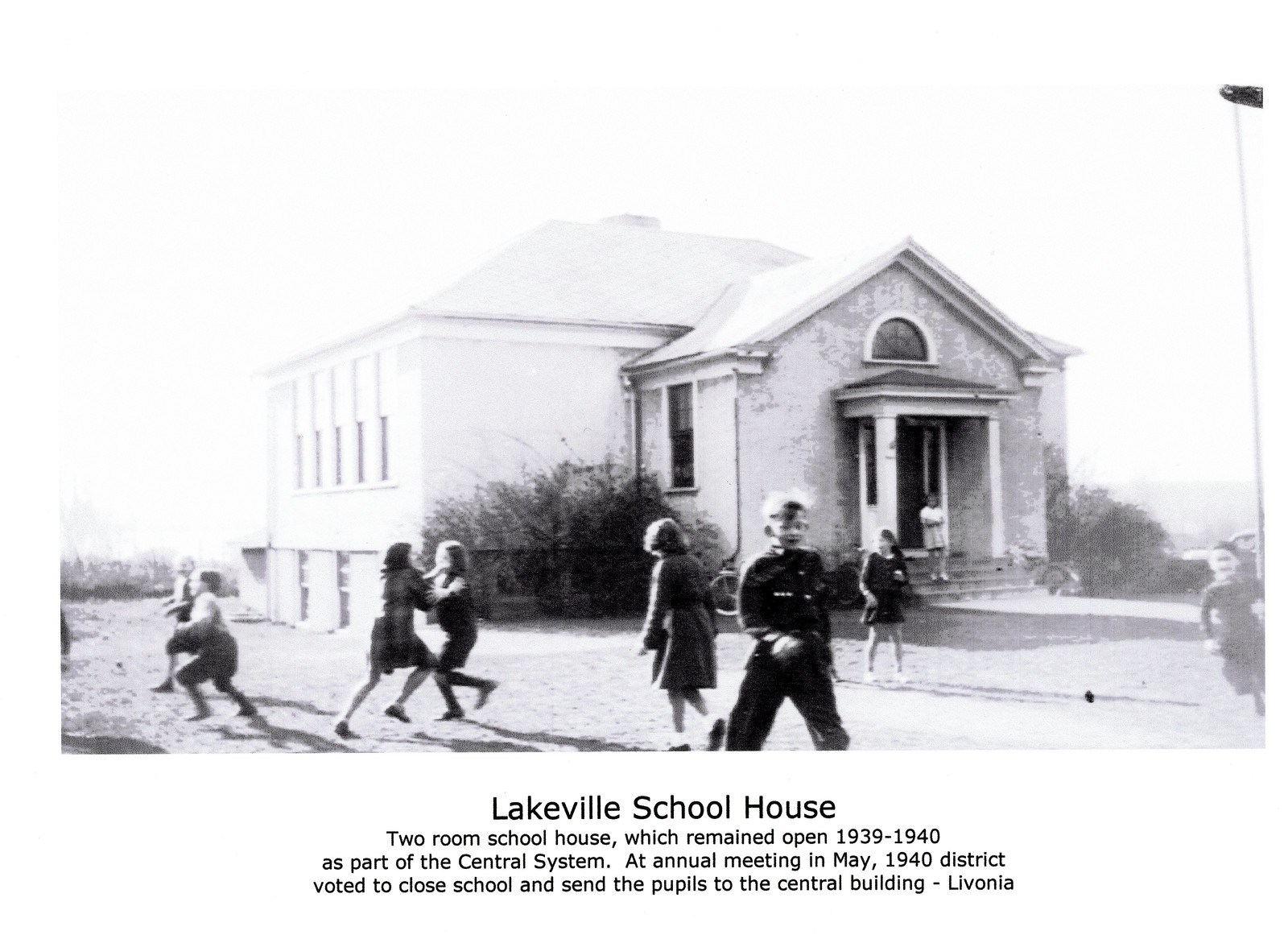This black-and-white photograph captures a moment in time at the Lakeville Schoolhouse, a two-room brick building that operated as part of the central system from 1939 to 1940. Below the image, text notes that during an annual meeting in May 1940, the district voted to close the school and transfer pupils to the central building in Livonia. The weathered photo shows the schoolhouse surrounded by bushes and shrubs. In the foreground, a group of about ten children, most of them girls in dresses and skirts typical of that era, are playing and running around in the schoolyard. One boy is seen standing on the steps of the school, facing and walking towards the camera. The white sky and overall condition of the image suggest it has endured the passage of time, adding a layer of historical context to this quaint, nostalgic scene.